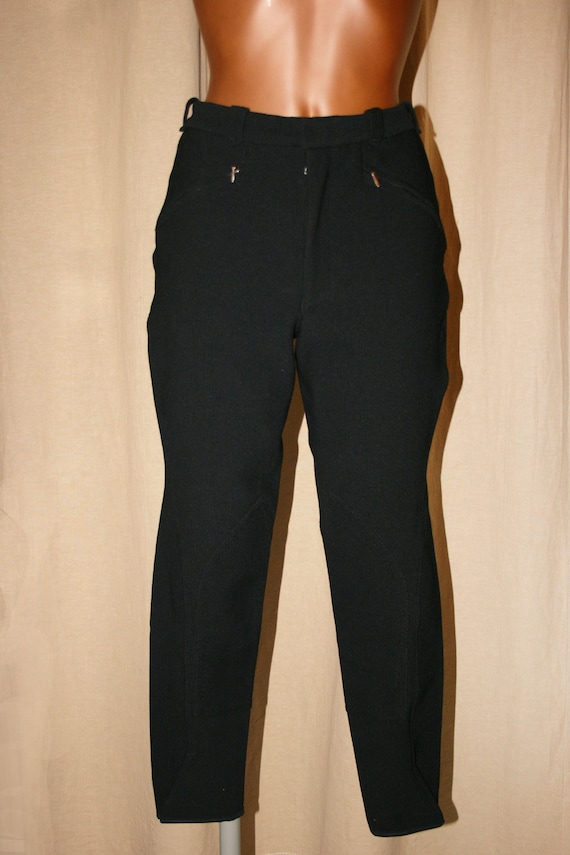The photograph features a rectangular, vertical image, approximately five inches high and three to four inches wide, taken indoors against a light camel-colored or tan curtain backdrop. The central focus of the image is the stomach and waist area of a shiny, bronze-colored or brown mannequin, mounted on a small white or silver metal pole. The mannequin is modeling a pair of black full-length pants that prominently occupy the center of the frame. These pants, which appear slightly too large for the mannequin's waist, have belt loops, a central zipper, and pockets on either side, each adorned with little zipper tabs. There is a subtle shadow effect on the right side of the pants. The pole affixing the mannequin is partially visible emerging from the bottom of the left pant leg, and the backdrop is simple, accentuating the mannequin and the black pants.